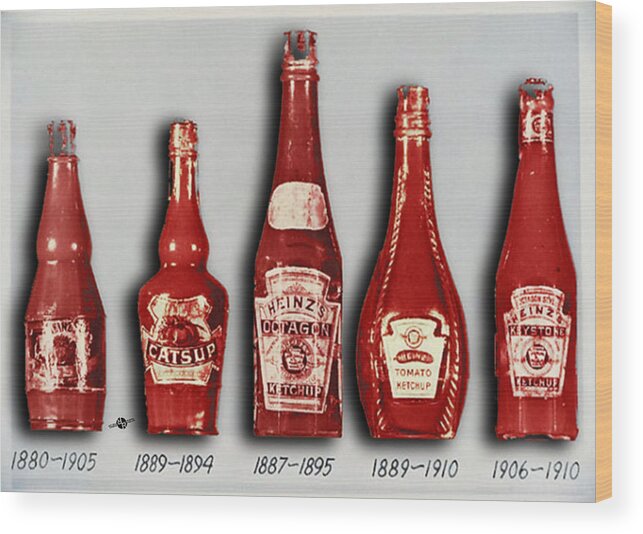The image depicts five bottles of ketchup arranged horizontally against a light grayish blue background, representing the evolution of ketchup packaging over time. From left to right:

1. The first bottle, a regular-sized ketchup bottle, partially reveals its label and is marked with the years 1880-1905.
2. The second bottle, similar in size, has a front label featuring the word "ketchup" and an image of a tomato, and is marked with the years 1889-1894.
3. The third bottle is slightly taller, with labels at the neck and main body, partially showing the word "Heinz." It is marked with the years 1887-1895.
4. The fourth bottle is a bit shorter and fatter than the Heinz bottle, featuring a white label with the words "tomato ketchup." It is marked with the years 1889-1910.
5. The fifth and last bottle, slightly skinnier than the previous one, also displays a label with "Heinz" and is marked with the years 1906-1910.

Overall, this image visually documents the progression and branding changes of Heinz ketchup bottles over several decades.